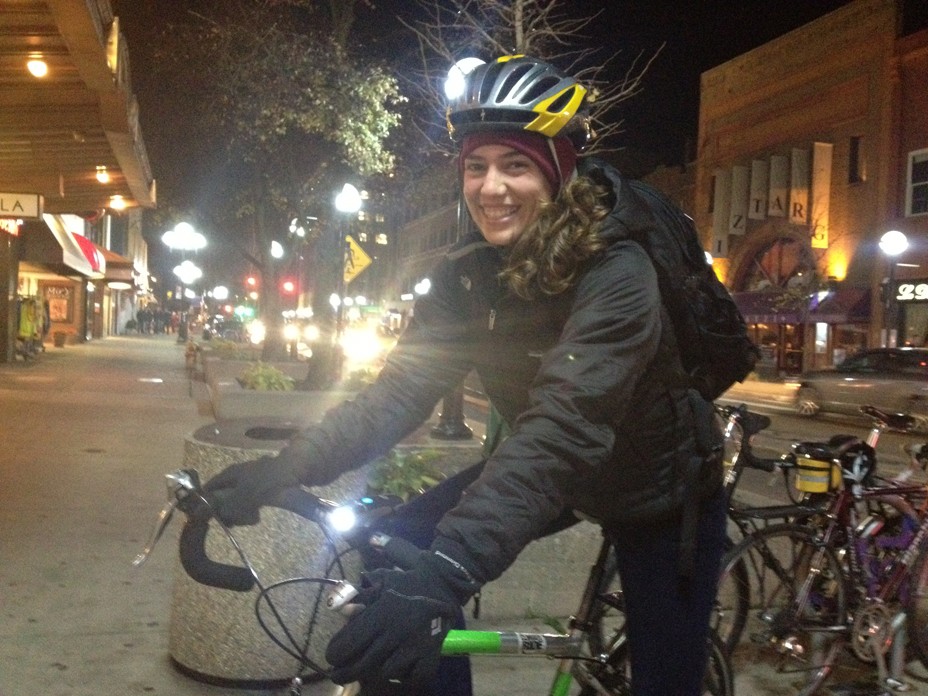The image captures a nighttime urban scene with a female cyclist in the forefront. She is donning a black and yellow helmet paired with a red hat, and she is smiling, revealing a fair complexion. Her brown curls cascade over her right shoulder in the image. She wears a black jacket, either navy blue or black pants, and black gloves. A black book bag is strapped to her back, adding to her casual yet sporty appearance. Her bicycle has a bright light mounted in the front-center, and the handles are black, with the frame showing a mix of silver and green hues. In the background, multiple bikes are parked, suggesting a busy area. Streetlights illuminate the scene alongside red traffic lights, indicating the presence of traffic. The sidewalk she is on is lined with stores, adding to the bustling city atmosphere.